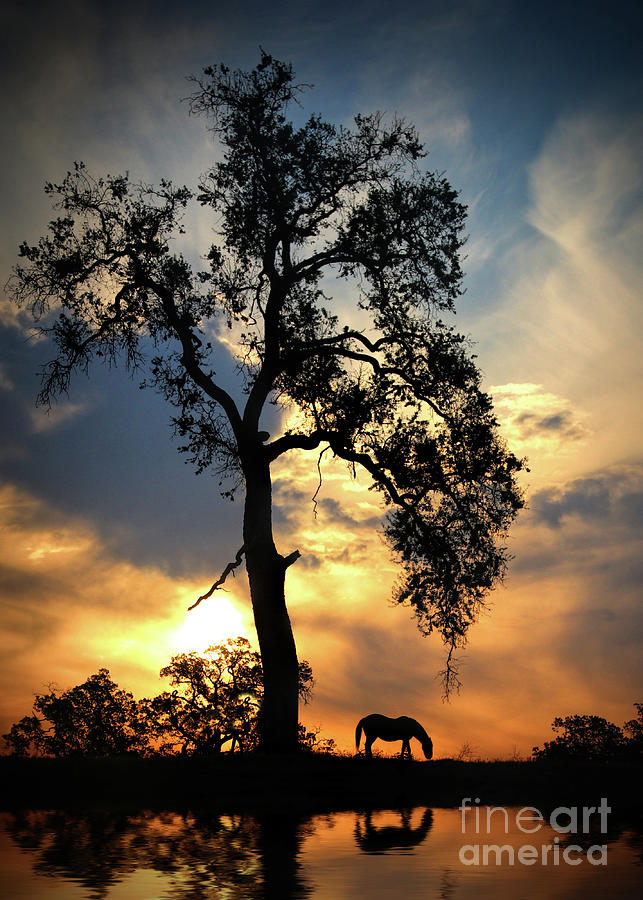The photograph captures a striking sunset scene dominated by the silhouette of a large, leaf-bare tree standing prominently near a calm body of water that mirrors the vivid hues of the evening sky. To the left of this central tree, smaller trees also punctuate the horizon in silhouette. On the right, a horse is seen with its head down, grazing, its dark form blending into the fading light. The sun, almost touching the horizon, illuminates the scene with an intense orange glow, and the sky above transitions from deep oranges and yellows near the horizon to blues and whites higher up, interspersed with dark gray clouds and wispy white cirrus clouds. The tranquil water in the foreground perfectly reflects the towering tree, the horse, and the rich array of sunset colors. In the bottom right corner, the faint text reads "Fine Art America," adding a subtle watermark to this serene and picturesque nature photograph.